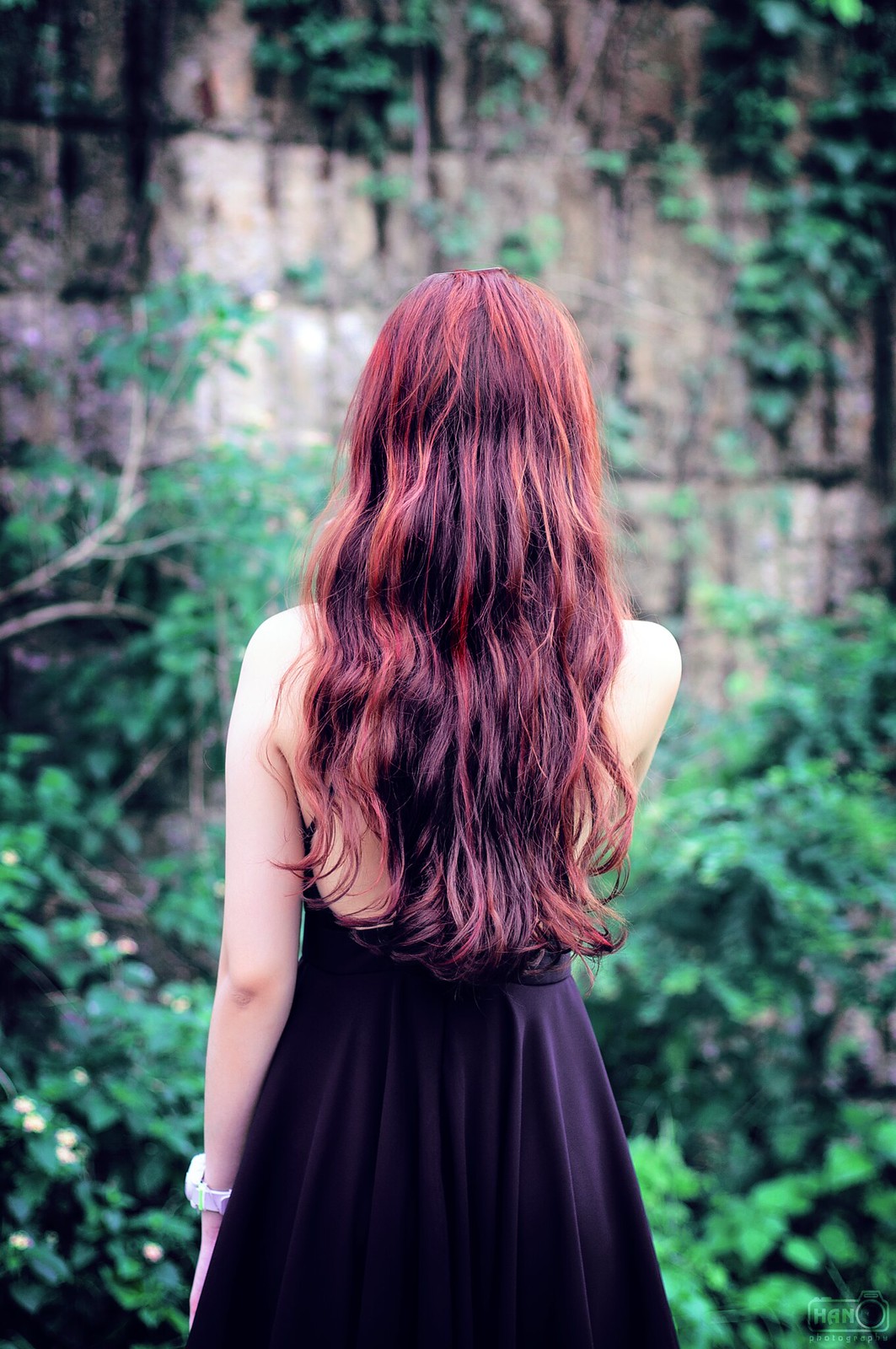In the photograph, a woman stands with her back to the camera, facing a sheer, out-of-focus cliff wall adorned with lush greenery. Her long, wavy hair, dyed red and brown, cascades below her shoulders. She wears a backless, sleeveless black dress that elegantly contrasts with the vibrant vegetation surrounding her. Her left wrist is adorned with a white wristwatch. The cliff wall, composed of light beige stone with darker edges, is abundantly covered in vines, leaves, and tree branches, adding rich textures to the background. The lower part of the image reveals dense greenery and bushes, contributing to the verdant ambiance of the scene. In the bottom right corner, a white watermark with the letters "HANO" and some illegible text is visible. One of her arms rests by her side while the other is positioned in front of her. The scene is captured outdoors during the day, with the main subject in sharp focus against the slightly blurred, verdant cliff backdrop.